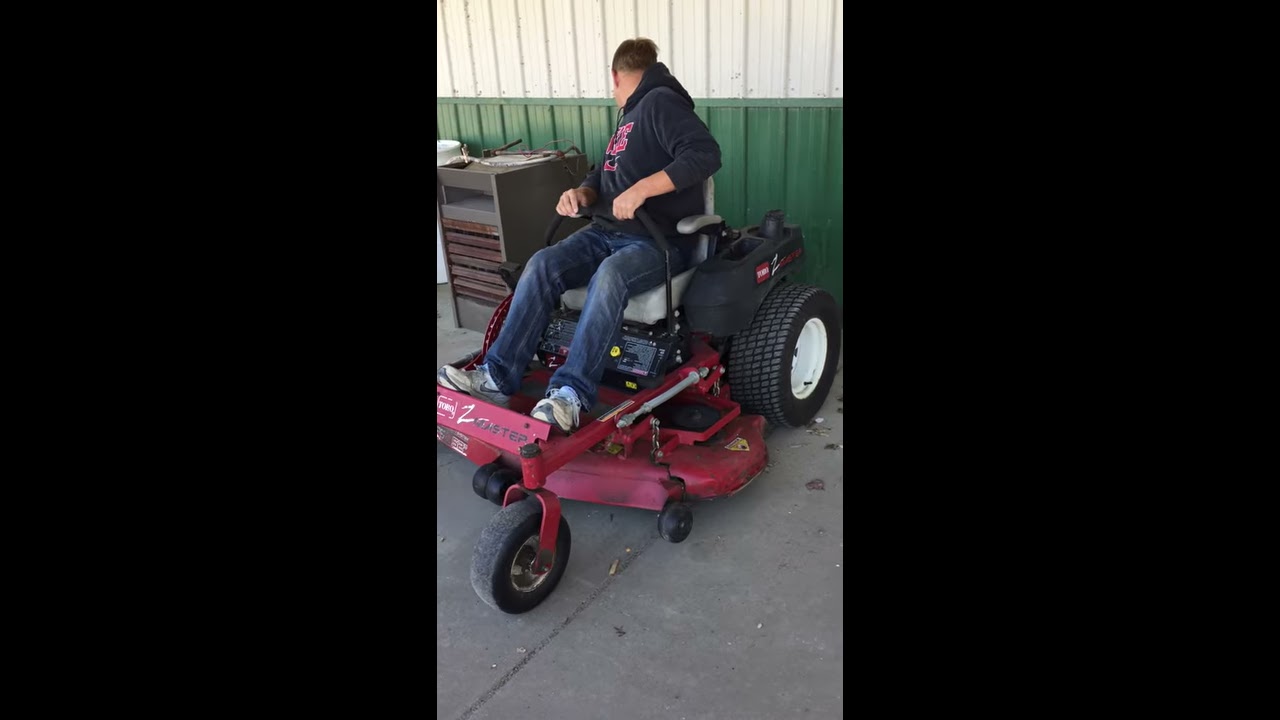In an outdoor setting reminiscent of a garage space, a white man with brown hair sits backward on a red zero-turn electric lawnmower. He is parked against a two-colored metal wall, painted green on the bottom half and white on the top half. He is dressed in a dark blue sweatshirt with red lettering, blue jeans, and white sneakers with blue and gray trim. The large rear wheels and smaller front wheels of the lawnmower, along with its gray and black seating area, are visible. On the mower's front, there are letters that appear to spell "HUSTEP" or "MUSTEP." To his left is an old, rusted tool cabinet with three or four shelves, and to his right is a brown shelving unit and another metallic structure. The ground beneath him is gray, and the photograph includes blacked-out blocks on both the left and right sides.